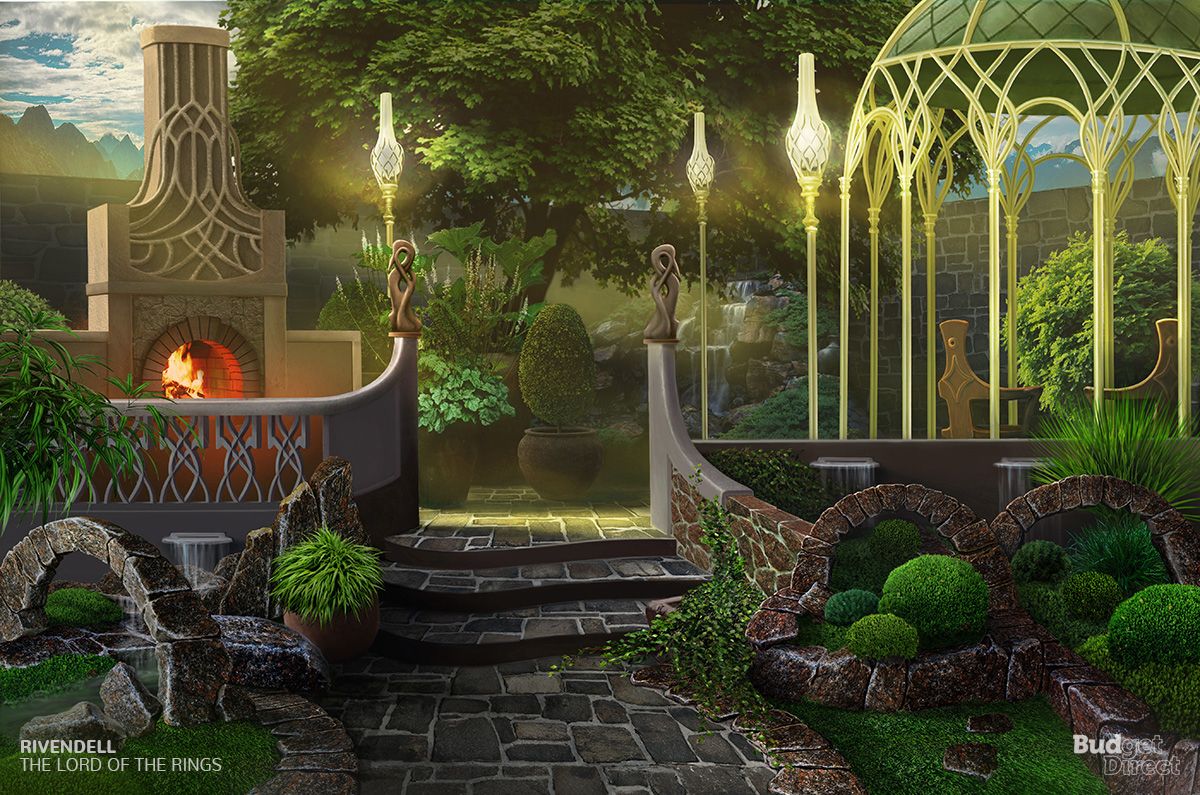This detailed 3D color illustration depicts a fantasy outdoor garden setting reminiscent of Rivendell from "The Lord of the Rings." The scene is enclosed by a stone brick wall and lit by soft lanterns on posts. Positioned centrally is a grand gazebo with a green-tiled, dome-shaped roof adorned with yellow latticework. Supported by vertical poles, the structure houses a couple of wooden chairs facing away. To the left, an elegant outdoor fireplace with a pointed chimney and a cream-colored trellis design exudes warmth with its yellow flames. Stone banisters and curved walls lead towards a set of grayish-brown flagstone steps at the center, inviting the viewer into the garden area. Sculpted gardens and arced walkways, outlined with bricks, flank either side of the scene. The background showcases dark green trees under a bright light blue sky dotted with white clouds. White text at the bottom left reads "Rivendell, the Lord of the Rings," pointing to the illustration’s fantasy inspiration.